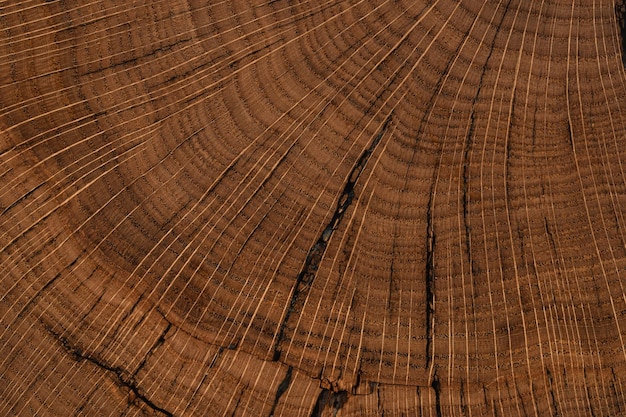This is a highly detailed, close-up photograph of the cross-section of a tree. The image, dominated by shades of brown ranging from light to dark reddish-brown, highlights the intricate wood grain and numerous growth rings that fan out from the top right corner across the entire frame. The rings, well-delineated in alternating lighter and darker tones, provide insight into the tree's age and the varying environmental conditions it experienced, such as years with scarce water and years with abundant water. The photo also captures several distinct cracks; the most prominent one runs from the bottom center, angling steeply to the right, revealing darker brown to black colors interspersed with small brown fragments. Smaller, similarly styled cracks branch out, adding depth and texture to the image. This close-up shot accentuates the natural beauty and complexity of the tree's interior, possibly even suggesting that it could be a section of a wooden table, though the complete absence of a background concentrates attention solely on the cross-section.